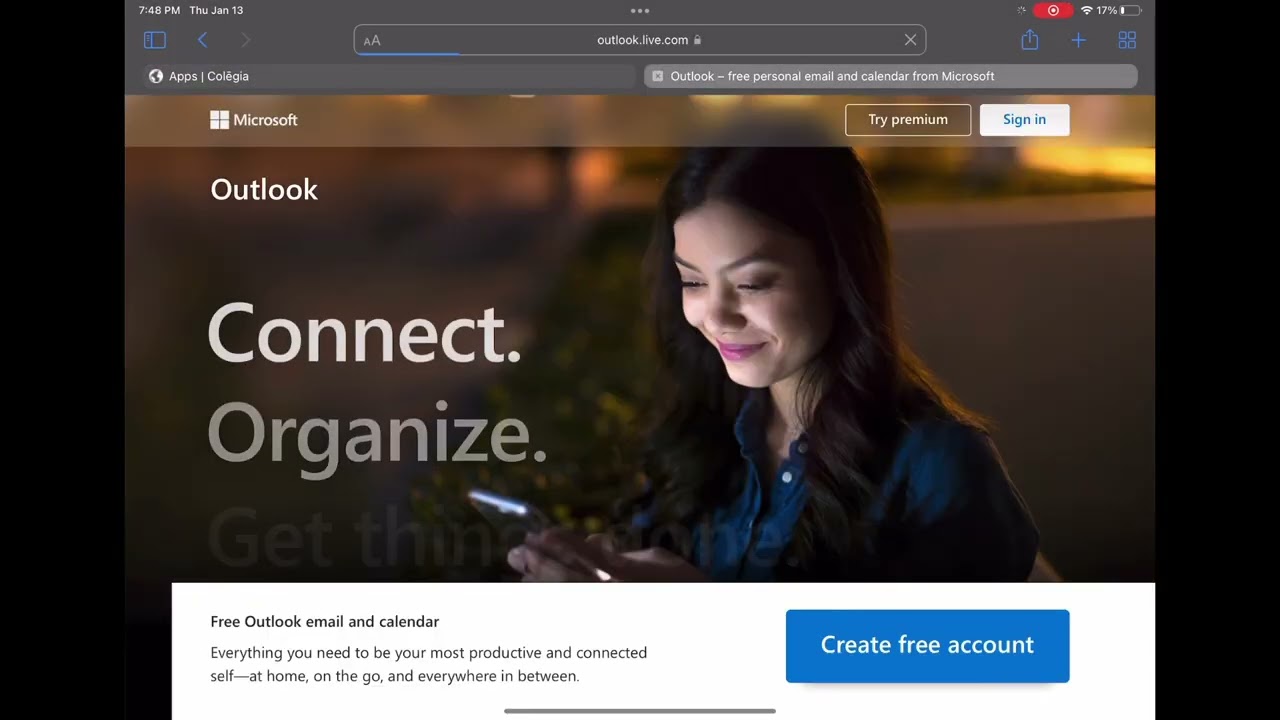The image displays the Outlook.live.com website interface, prominently featuring a search bar at the top. The navigation area is reminiscent of an Apple iPad with its sleek design. In the top left corner, the interface shows the date and time, specifically Thursday, January 13th. In the top right corner, there is a red recording icon, a Wi-Fi symbol, and a low battery indicator displaying 17%. Below these, a blue arrow pointing left and a gray arrow pointing right are visible.

On the right-hand side of the interface, there are several icons: a bookmark, a plus sign, and a grid of four blocks. Below these icons, two tabs are visible. The left tab, labeled "Apps Collegia," and the right tab, labeled "Outlook - free personal email and calendar from Microsoft."

Further down the page, there is an image of a woman in a blue shirt, smiling while looking at her phone. Above her image are the words "Microsoft" and two buttons labeled "Try Premium" and "Sign In." Below the image, large text reads "Outlook," followed by the tagline "Connect. Organize."

A white box beneath this text contains the phrase "Free Outlook email and calendar, everything you need to be your most productive and connected self, at home, on the go, and everywhere in between." Lastly, there is a blue button at the bottom of the box that says "Create Free Account."